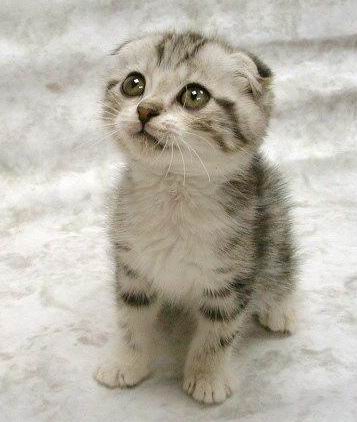A captivating image of a small striped kitten dominates the frame, showcasing its delicate black, gray, and light brown fur pattern. The kitten, with its wide, expressive eyes, gazes up towards the upper left-hand corner, creating a sense of curiosity and innocence. Its tiny whiskers and paws are clearly visible, adding to its endearing and vulnerable appearance. The background is plain and unobtrusive, making it ideal for adding text or additional elements to the image. This simplicity draws attention to the kitten, who seems to embody the sympathetic and relatable qualities often associated with popular internet memes. The legacy of cats in digital culture, notably proliferated by anonymous groups embedding hidden codes in cat images over a decade ago, is evident in this picture. Today, such images continue to resonate, offering a canvas for shared emotions and communal expressions.